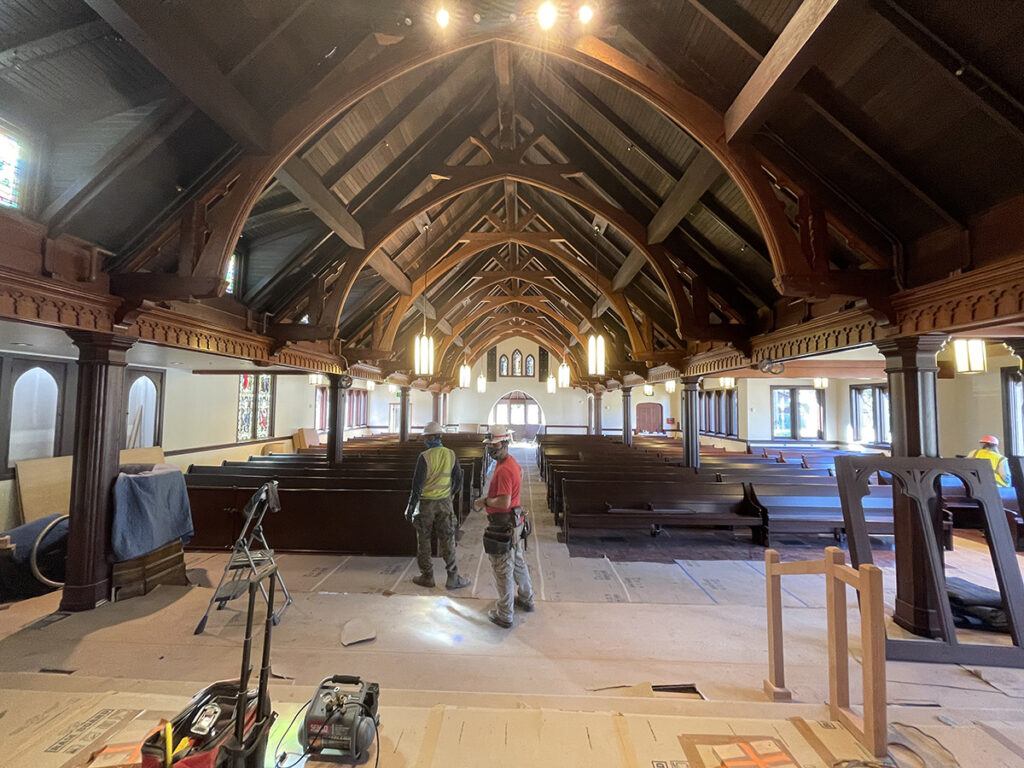The photograph depicts the interior of a church undergoing significant construction. The perspective is from the altar, looking down a central aisle that divides two rows of dark-colored pews. The church features elegant architectural details, including wooden arches with hanging lights and a triangular ceiling adorned with stained glass windows on both the upper and lower sections.

In the near foreground, unfinished wood flooring contrasts with the concrete-like surface of the aisle, which is taped off in various places. There are tools scattered around, including what appears to be a sander or saw on the left side, with more equipment nearby. On the left side of the photo, scaffolding and an uninstalled window frame are evident, hinting at ongoing restoration work.

Two construction workers stand prominently in the center of the image. The worker on the left, identifiable by his yellow construction vest and white hard hat, is turned away from the camera. The worker on the right, dressed in a red shirt and gray pants, is also wearing a hard hat and appears to be looking to his left. Both workers are equipped with tool belts and are engaged in floor installation.

In the background, multiple sets of pews are divided by pillars, and a rounded opening allows light to filter into the space. The detailed wood rafters create a vaulted effect, giving the ceiling a pointed central peak. Overall, the scene captures the intricate process of the church's renovation, with numerous construction elements meticulously placed throughout the space.